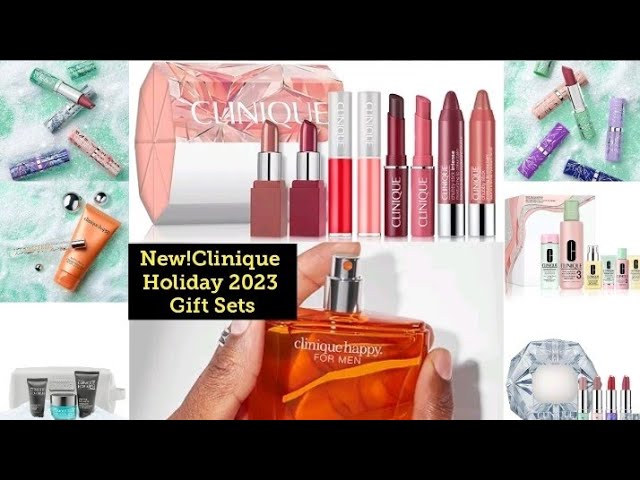The image is an advertisement for Clinique's new Holiday 2023 gift sets. It features a white background with a one-inch thick black border at the top and bottom. Inside the image, towards the middle left, there's a black square with yellow text that reads "New Clinique's Holiday 2023 Gift Sets." Surrounding this central text block are various product images. 

To the left, there's a green and white sandy background displaying items like lipstick, a face cream, and silver balls. The left bottom corner features a bottle containing blue liquid with a silver cap, as well as some squeeze bottles. At the top center, several different shades of lipstick are displayed next to a Clinique paper lantern. In the top right, lipsticks are laid out on a green and white glittery or sandy surface. Below this, there are green, red, and yellow bottles with writing on them and different colored caps, including green, red, and silver. The very center of the image prominently displays Clinique Happy for Men cologne in an orange bottle.